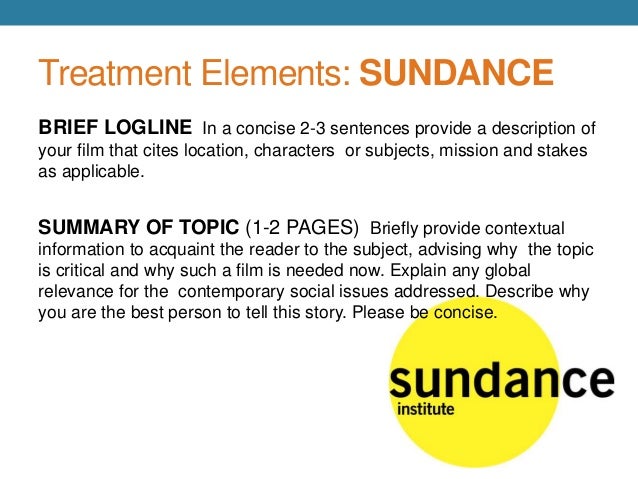The image is a text-based guideline for submitting a film to the Sundance Film Festival, featuring a horizontal dark blue line at the very top on a white background. Just below the line, it reads "Treatment Elements: Sundance," with "Sundance" in slightly bolder and darker orange, while "Treatment Elements" is a lighter orange. In black text underneath, it instructs the user to provide a "Brief Logline" in two to three concise sentences, describing the film’s location, characters, subjects, mission, and stakes. Following this direction, the next section titled "Summary of Topic," advises filmmakers to briefly provide one to two pages of contextual information to acquaint the reader with the subject, explaining why the topic is critical and relevant to contemporary social issues, and why the filmmaker is the best person to tell the story. At the bottom right of the image, there is a yellow circle with the text "Sundance Institute" in black lettering overlapping the circle, representing the Sundance Institute logo.